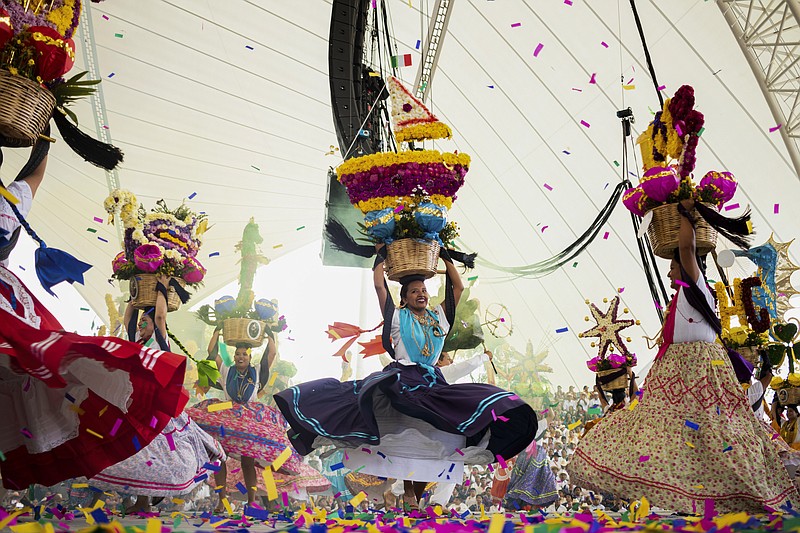The image depicts an outdoor celebration, likely Mexican, under a large white canopy. It is a horizontally aligned rectangular photograph taken on a somewhat dreary day. The scene is filled with vibrant colors, including red, yellow, pink, purple, blue, beige, black, brown, and tan, adding life to the festive atmosphere. In the foreground, there are three prominent women, each dressed in long, flowing skirts that give the impression of twirling. The central woman wears a navy skirt with lighter blue stripes at the bottom. She appears to be sitting or possibly doing a split, holding a wicker basket full of elaborate floral designs akin to a sailboat above her head. To her right is another woman in a gold, red, or dark pink patterned skirt and white top, also lifting a wicker basket adorned with flowers and other decorative objects. To the left stands a woman in a red and white striped skirt with a white top, similarly holding a basket filled with decorations. Behind her, another woman can be seen partially, wearing a hat with a huge floral star. Confetti in red, blue, yellow, and pink hues covers the ground and is visibly falling through the air, enhancing the celebratory mood. The background features horizontal white wooden boards reminiscent of a ship's side, adding depth to the scene. The women seem to be dancing, surrounded by many others in the background, all contributing to the lively and joyous ambiance.